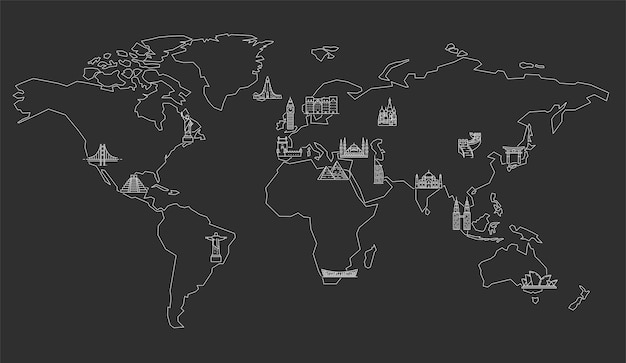The image showcases a world map with a matte black or very dark charcoal gray background, and all continents are outlined in stark white thin lines. Scattered across the continents are intricate white drawings of cultural landmarks, detailed without any labels or text. Each continent features iconic monuments: the Golden Gate Bridge in California, the Statue of Liberty, and the pyramids of Teotihuacan in Mexico on the North American continent; the Jesus statue in São Paulo, Brazil in South America; Big Ben in London, the Alhambra in Spain, and other famous structures in Europe; the pyramids in Egypt representing Africa; the Sydney Harbour in Australia; the Great Wall of China and the notable tori gates of Japan in Asia. The entire map maintains a horizontal rectangular orientation, offering a detailed and artistic representation of global landmarks through minimalist yet precise white line art on a dark backdrop.